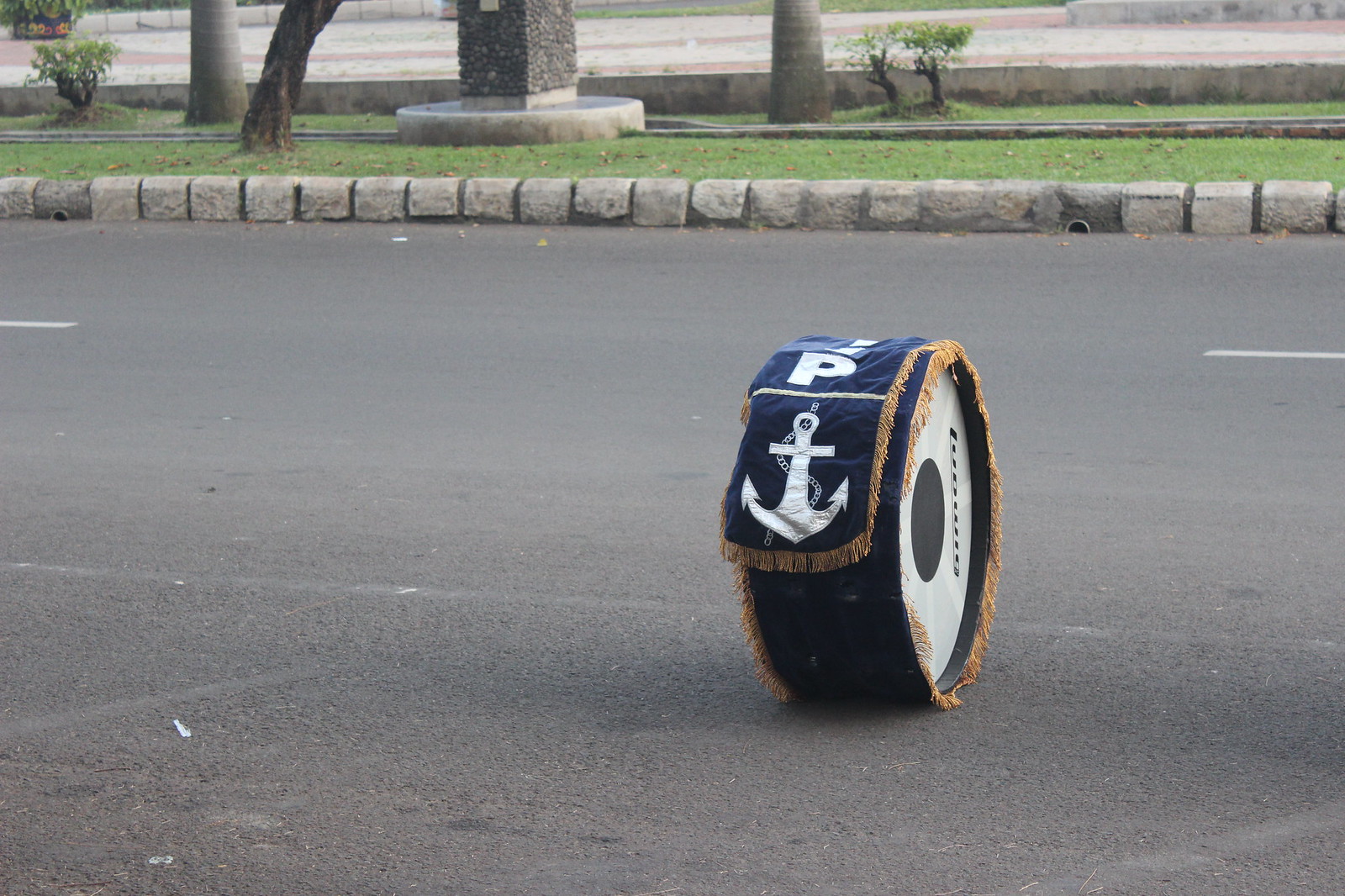In the image, we see a scene set outdoors on a road with a nearby sidewalk bordered by a curb featuring gray bricks. The prominent focus of the image is a large, wheel-shaped object situated in the middle of the road. This object resembles a drum, possibly a part of a drum kit used in marching bands, suggesting it might be for a naval procession or parade. It is covered with a velvety navy blue banner that features gold-colored tassels along its edges. The banner has an embroidered design including a white anchor with a chain, along with white lettering that includes an "IP" and another barely recognizable inscription.

The drum-like object has a round and light gray spindle with the name "LUDWIG" inscribed on it in black letters. The road beneath it is gray with some dashed white lines and a solid, albeit faded, white line. In the background, the scene includes trees with visible stumps and patches of grass. Additionally, there is a side platform, potentially holding a water fountain, highlighted by gray and white rocks, and a distant sidewalk with a distinct red and white pattern.